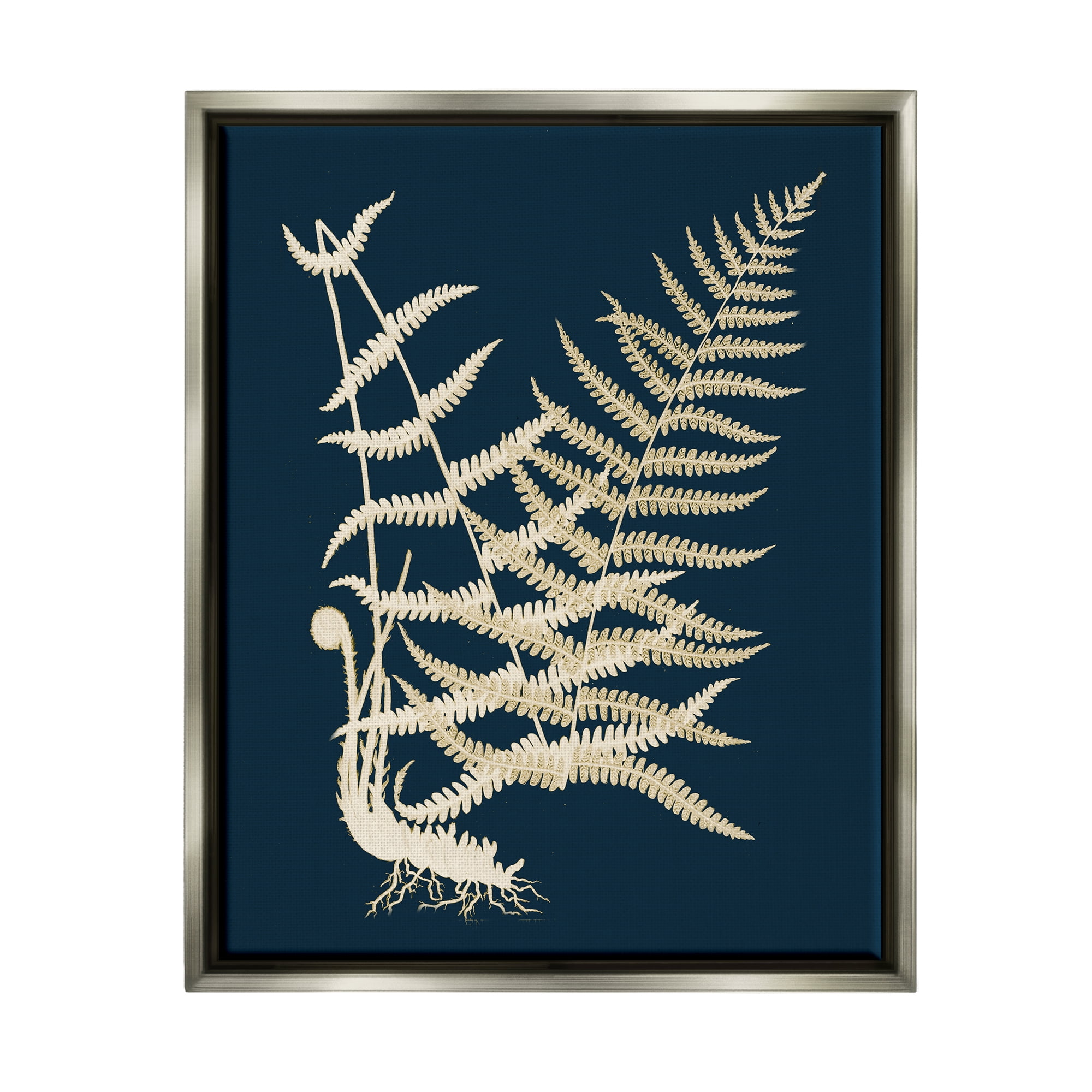This image showcases a beautifully framed artwork featuring pressed leaf art. Housed in a silver metal frame with a black inner lining, the piece presents a striking composition on a navy blue canvas. The artwork displays two main fern leaves with roots extending from the bottom, giving a sense of depth and texture. The leaf on the left is partially incomplete, missing several leaflets, whereas the leaf on the right is fully intact. The fern leaves, in shades of tan with a whitish hue, appear to be meticulously dried and pressed, indicating a delicate preservation process. The detailed black border enhances the contrast between the vivid navy backdrop and the intricate patterns of the fern leaves, making it a compelling and visually arresting piece of wall art.